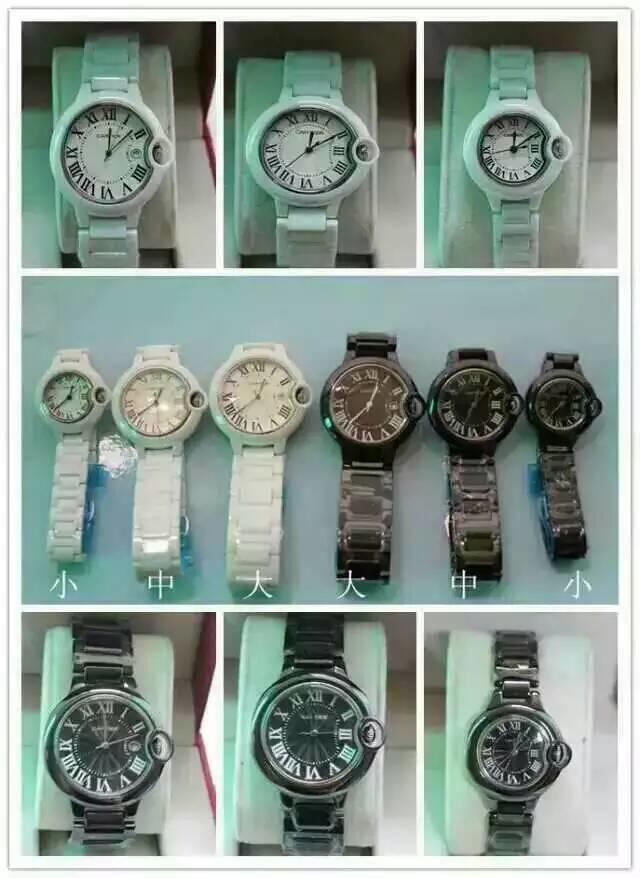The image showcases an organized display of watches arranged in three distinct rows. 

- The top row features three watches with pale green straps and white faces, each accentuated with Roman numerals.
- The second row exhibits a unique arrangement: three black watches showing only their lower bands are lined up vertically, while on their left side, three more pale green watches with white faces and Roman numerals are displayed horizontally. Beneath each of the six watches in this row, there are inscriptions resembling Asian characters.
- In the third row, there are three watches with sleek black faces and elegant silver bands, also displaying Roman numerals.

The meticulous arrangement highlights the variations in design and cultural elements displayed in the timepieces.